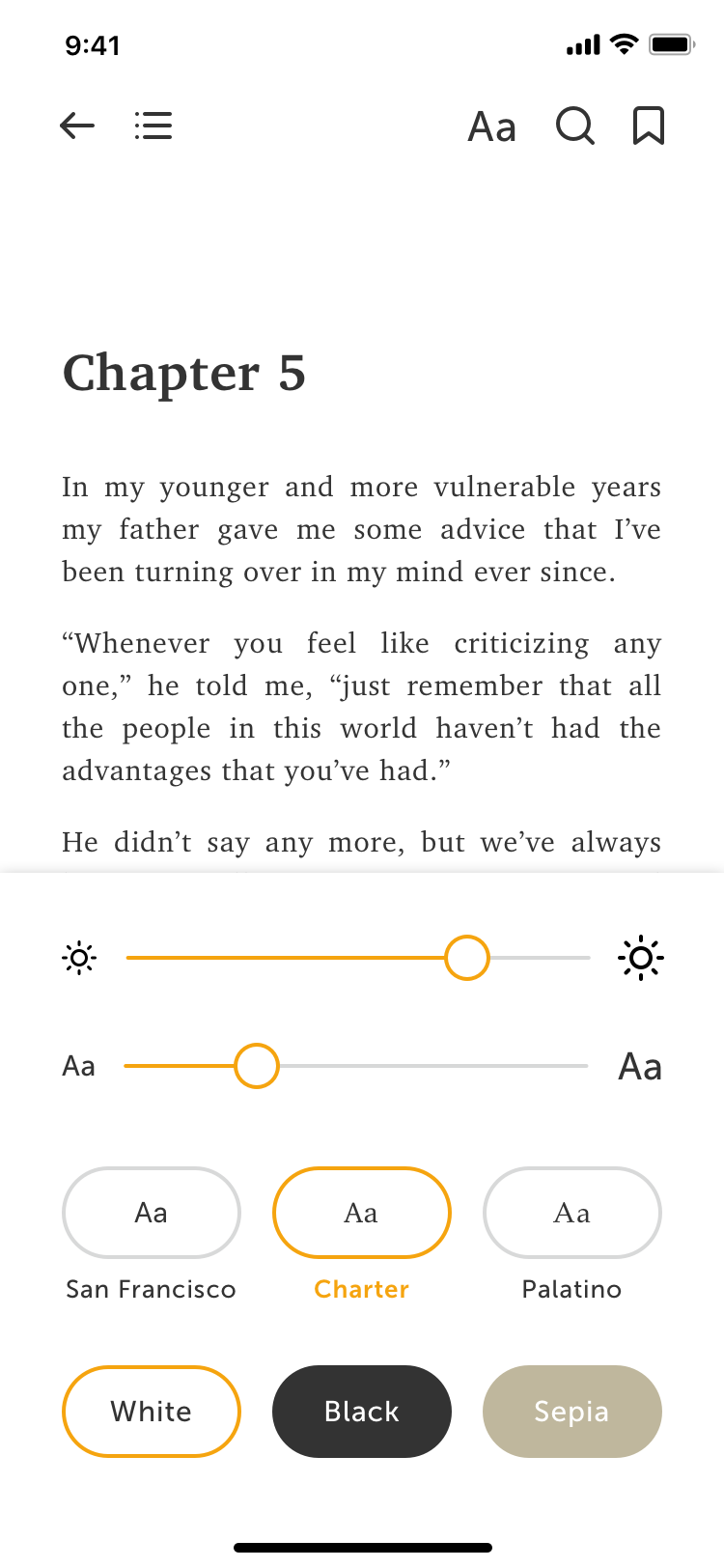Here is the cleaned-up and detailed descriptive caption:

---

This image is a screenshot from an e-reader, likely a Kindle, displaying a passage from a book. The time shown on the device is 9:41 AM, and it indicates full battery, full Wi-Fi, and full cell service. In the upper portion of the screen, there are navigation icons including a back arrow, a menu symbol, and text formatting options denoted by a large 'A' and a small 'a'. There are additional icons: a microphone, a magnifying glass for search, and a bookmark.

The main content area displays significant white space. Prominently, the title "Chapter Five" appears in large black letters. Below, in slightly smaller black text, there's the opening line of the chapter: "In my younger and more vulnerable years, my father gave me some advice that I've been turning over in my mind ever since. 'Whenever you feel like criticizing anyone,' he told me, 'just remember that all the people in this world haven't had the advantages that you've had.'" The text is cut off by a menu bar, which is partially visible at the bottom.

The menu bar also features a brightness control slider, currently set at about 75%. Below that, text size adjustment options are indicated by a small 'a' and a large 'A'. The text size is adjusted to approximately 25% of the slider. Additionally, there are options for different fonts, including San Francisco, Charter, and Palatino, as well as color schemes such as white, black, and sepia. 

---